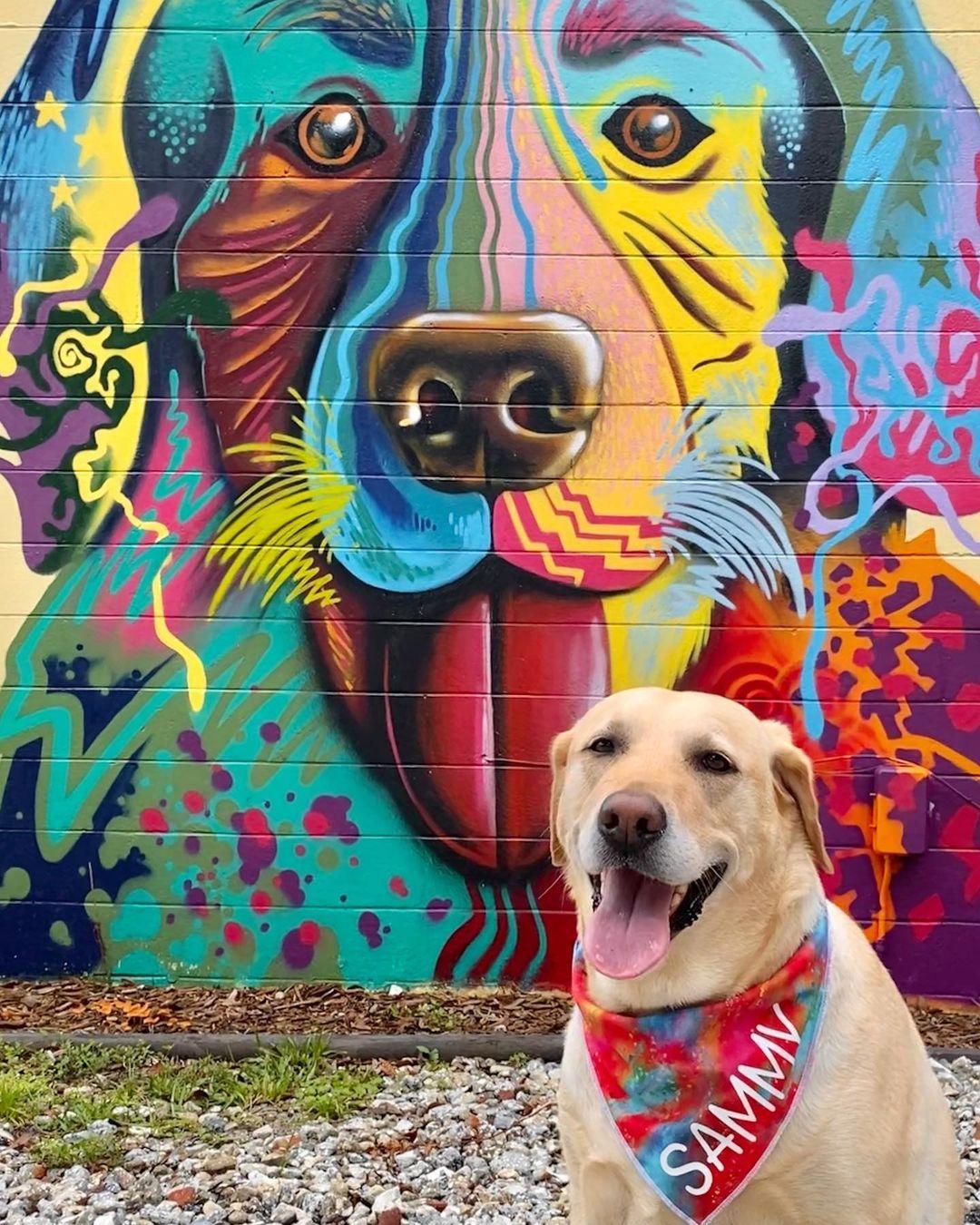This vibrant color photograph captures a joyful yellow Labrador-like dog named Sammy, identifiable by the white letters spelling "Sammy" on his tie-dye handkerchief. Sammy's short-haired coat is a very light yellowish-tan, and his happy demeanor is accentuated by his open mouth and tongue hanging out. The colorful handkerchief around his neck features red, blue, and orange hues. Behind Sammy, the setting reveals a mix of grass, soil, and gray rocks, leading up to a large wall adorned with a stunning piece of professional graffiti art. The mural depicts a psychedelic version of Sammy's likeness in a spectrum of vivid colors including blues, purples, pinks, reds, oranges, magentas, and aqua. The graffiti dog mirrors Sammy's expression, with its own tongue out and an array of polka dots and vibrantly painted whiskers. The overall scene seamlessly blends the real and the artistic, highlighting the spirited character of Sammy in both his physical form and his colorful doppelganger.